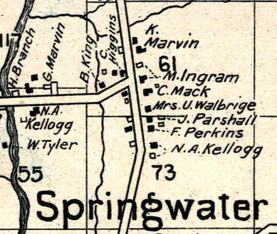The image portrays a detailed section of an old map characterized by an off-yellow, aged background with a grid of fine black lines. Dominating the bottom of the image is the bold text "spring water." A curving road or river traverses the left side from top to bottom, labeled with various identifiers including "55" and "117." Along this path, places and landmarks are annotated with names like Kellogg, W. Tyler, H. Branch, G. Marvin, K. Marvin, M. Ingram, C. Mack, and Mrs. U. Walbridge. The map also features what appear to be black blocks symbolizing buildings or houses next to which these names are inscribed. Another prominent element includes a stream cutting through the middle of the map, enhancing the aged and intricate nature of this historical cartographic detail.